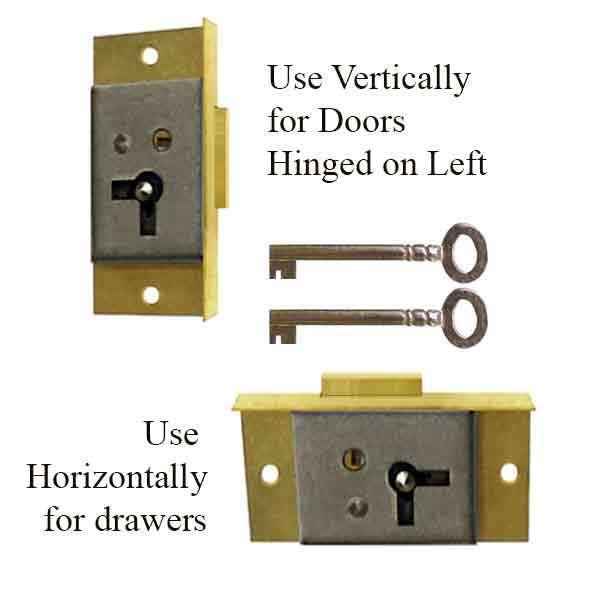This detailed image showcases an information sheet about locks and keys. The central focus features two identical locks and two identical keys. Both keys are a perfect match for the corresponding locks displayed. 

The text on the image is strategically placed at the top right and bottom left corners, written in dark brown letters. Specific instructions on the positioning of the locks are provided: they are to be used vertically for doors with hinges on the left (as noted in the top right) and horizontally for drawers (as indicated on the bottom left).

The locks themselves are composed of a gold-tone plate featuring a gray metal assembly positioned behind it. One side of each lock includes a flange with a hole. This is where the lock mechanism extends, allowing it to fit securely into a door or a drawer crevice.